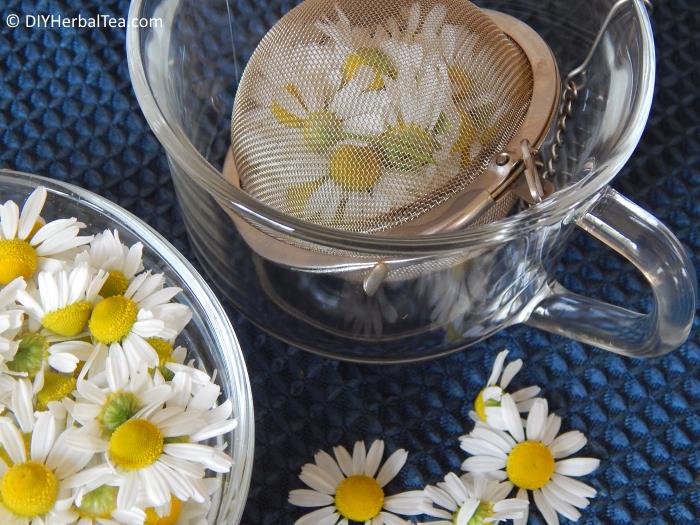The image showcases a beautifully arranged tea set focused on DIY herbal tea-making with daisies. In the upper left corner, the website "DIYHerbalTea.com" is prominently displayed. The set includes two main glass containers: a clear glass bowl on the bottom left brimming with daisy heads—white petals with yellow centers—and a clear glass teacup with a small handle on the bottom right. This teacup contains a mesh orb tea infuser filled with more daisy blossoms, although it lacks water at the moment. Additionally, three daisy flowers are elegantly placed on a blue, textured cloth surface beneath the teacup, enhancing the aesthetic. The overall arrangement cleverly combines elements for both practical tea brewing and visual appeal.